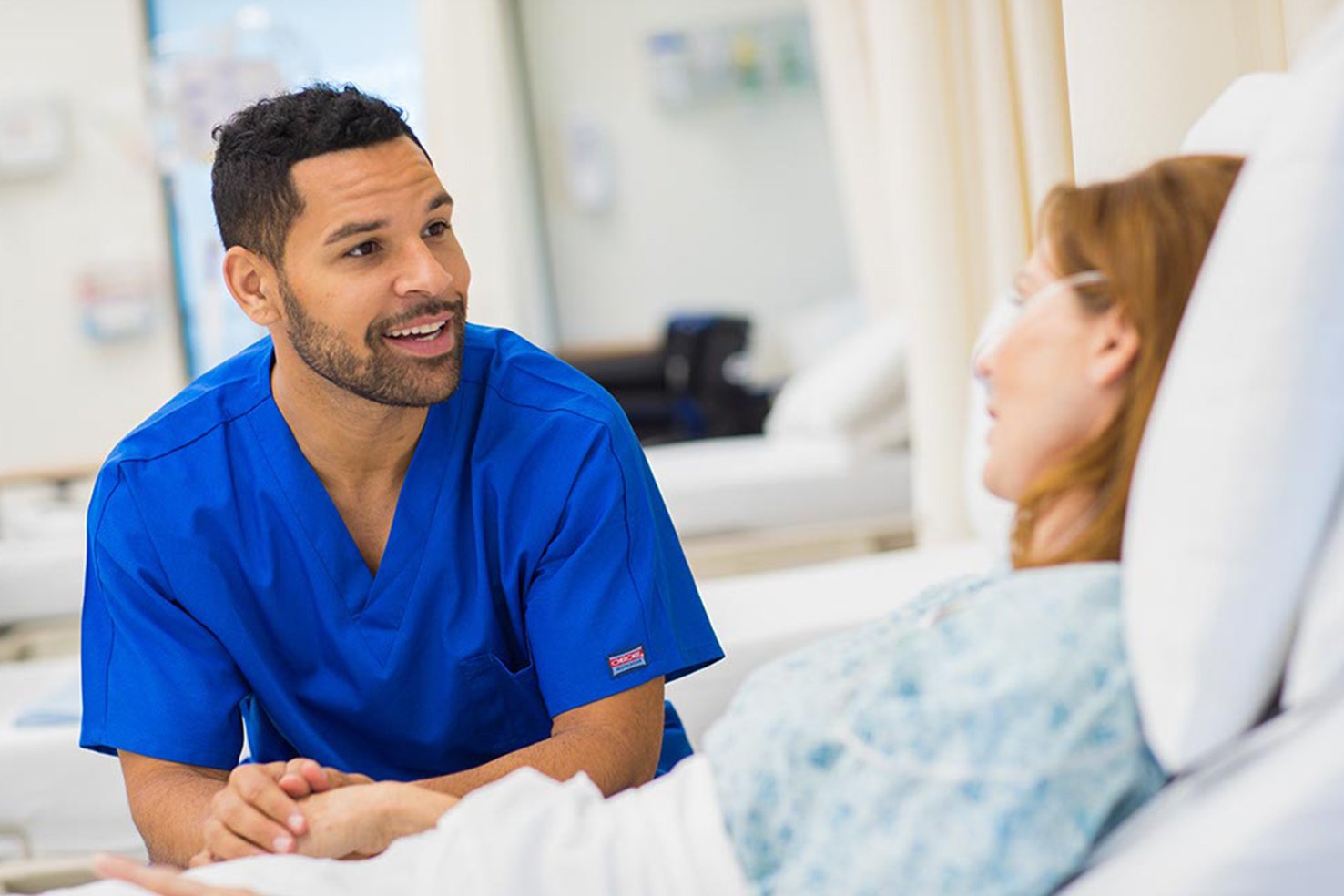The image captures a man, likely a healthcare professional given his bright new blue scrubs with a logo tag on the left sleeve, deeply engaged with a woman lying in a hospital bed. The man, who has dark short hair and a close-cut beard, is clasping the woman's right hand in both of his and smiling, perhaps discussing her condition or providing comfort. His mouth is slightly open, indicating he might be speaking to her. The woman, who has shoulder-length brown hair with subtle auburn highlights, is partially obscured and slightly out of focus. She appears young and wears a hospital gown with white sheets and blankets pulled up to her midsection. An oxygen tube extends across her face, suggesting she is receiving supplemental oxygen. The hospital setting includes white curtains, another bed, and a window in the background. Overall, the image conveys a sense of care and attentiveness.